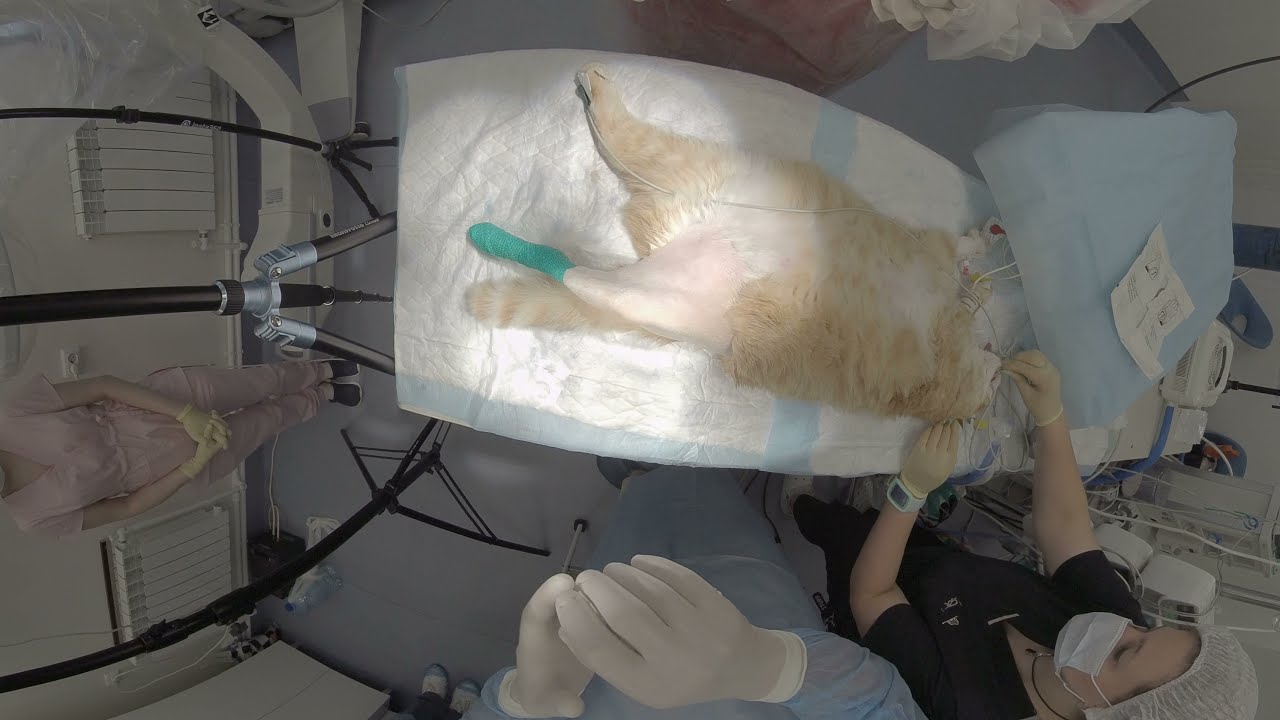The image depicts a point-of-view shot from a veterinarian's perspective, centered on a large, fluffy yellow cat with white fur on its stomach and chin, lying on its back on an operating table. The cat's left leg is completely shaved and wrapped in bandages, hinting at a recent surgery, while its furry tail pokes out from beneath it. Wires are attached to the cat's right leg, monitoring its vitals, and a tube is being positioned into the cat's mouth by a vet in blue scrubs and white latex gloves. Opposite the vet, a nurse in dark scrubs, a surgical mask, and headgear is gently holding the cat's head. In the background, an overhead light illuminates the scene, casting a focused glow on the cat's lower body. To the far left of the image, a woman in pink scrubs and yellow gloves stands attentively, her face partially outside the frame. Surrounding the operating table are various medical instruments, tubes, and equipment, reinforcing the clinical setting.